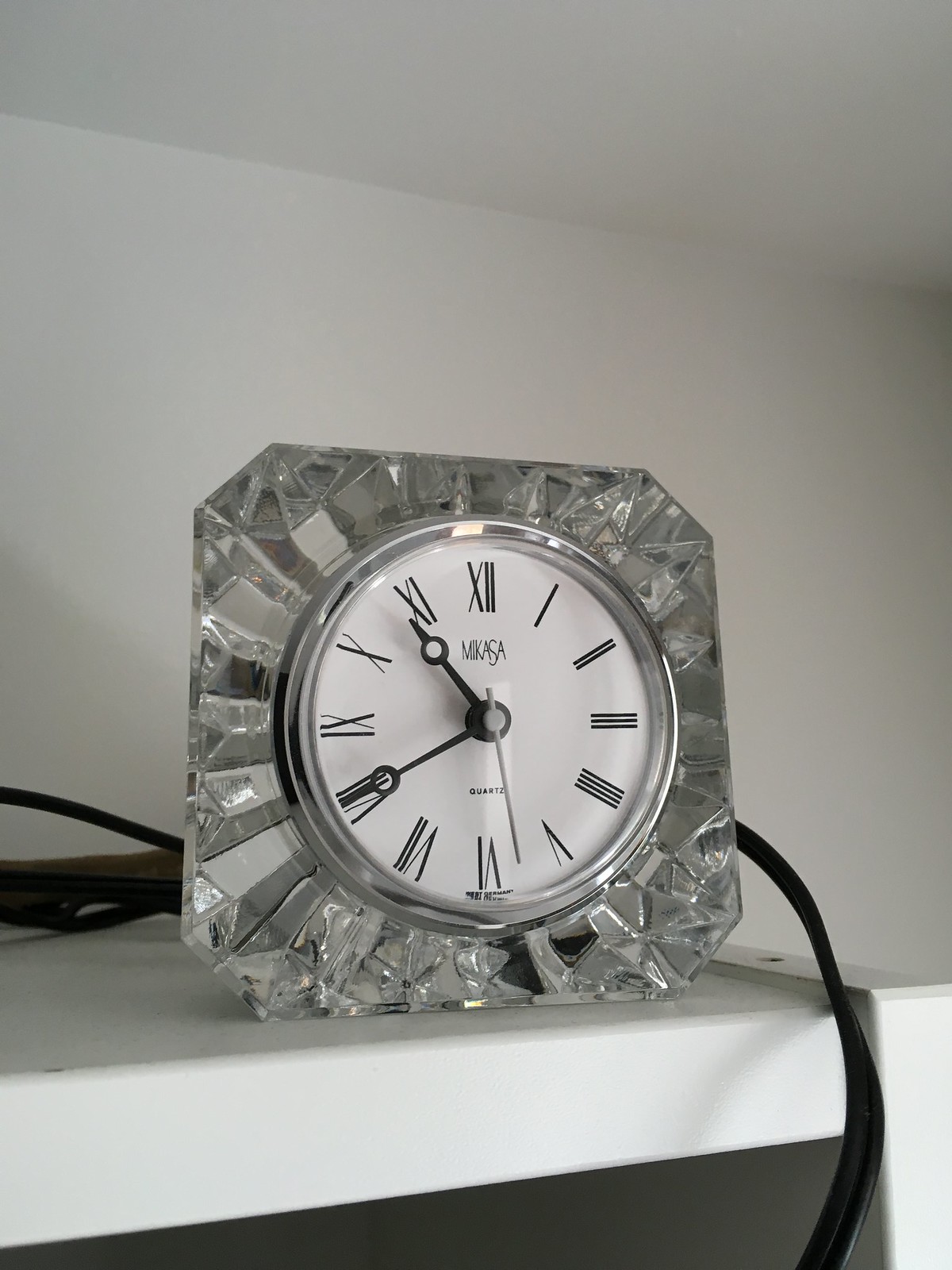This image features a vintage Mikasa clock positioned on a pristine white shelf, set against an all-white background. The clock boasts a crystal, ashtray-like square body, encasing a chrome-edged circular white face. Its time is marked by black Roman numerals I through XII, with black hour and minute hands and a lighter-colored second hand. The "Mikasa" logo is discernible beneath the 12 o'clock mark. Reflecting ambient light, the crystal surface captures glimmers from the room. Surrounding the clock are numerous black wires—one trailing down the front of the shelf and others bundled behind—suggesting they belong to equipment other than the clock. Shadows cast on the white backdrop enhance the clock's elegant yet utilitarian presence.